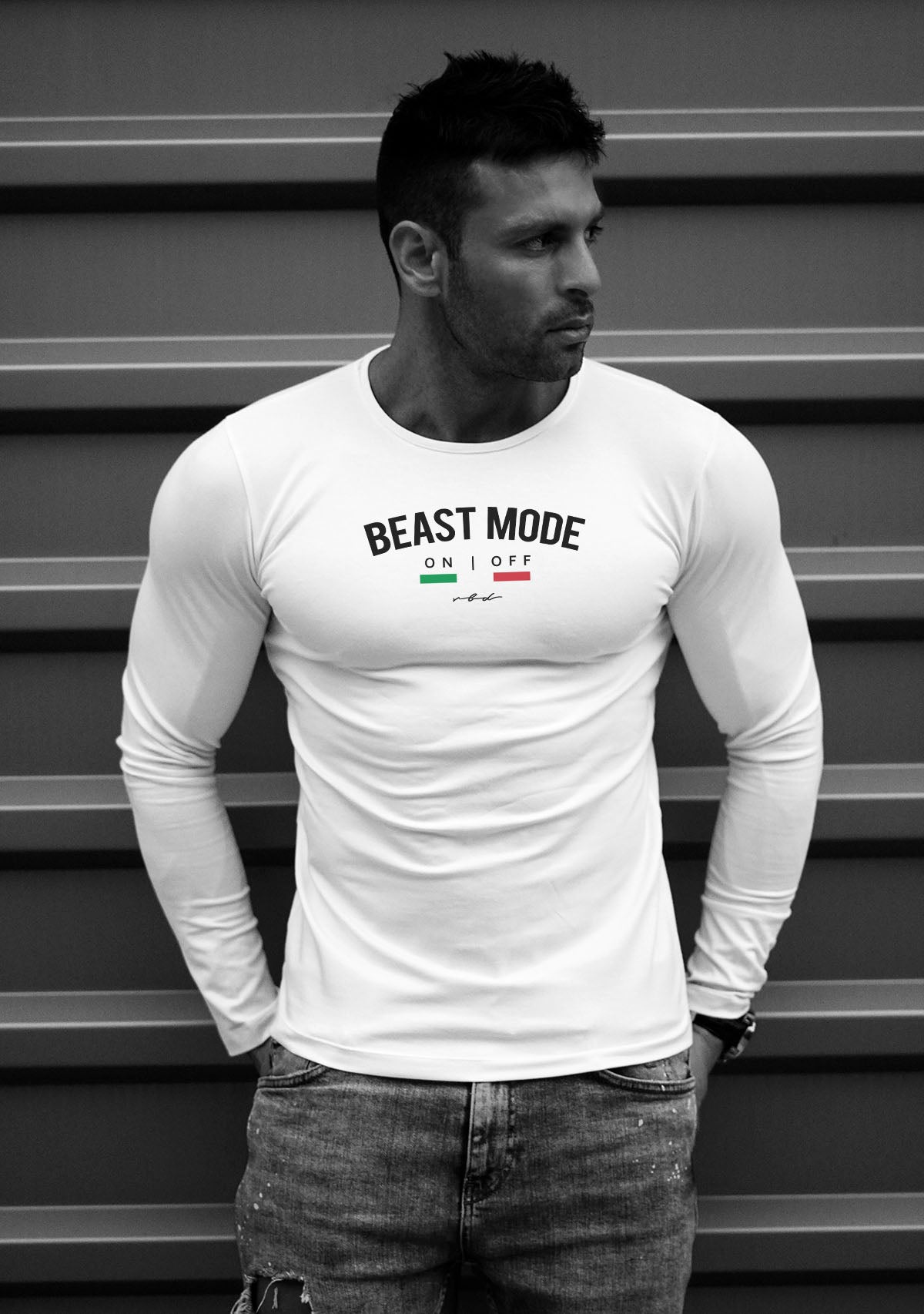The photograph is predominantly black and white, featuring a muscular man, possibly of Latino or Italian descent, with short black hair and a medium complexion. He is the central focus of the image, standing in the middle and looking to his left (the picture’s right). He dons a somewhat loose-fitting, long-sleeve white t-shirt with bold, black capital letters that read "BEAST MODE." Below the text, there’s a green bar under the word "ON" and a red bar under the word "OFF," with a tiny inscription or logo underneath that is too small to discern. He is also wearing dark, likely blue jeans, though there's some ambiguity about whether they are cut-off shorts or long jeans. His hands are positioned behind him, possibly in his back pockets, and he is accessorized with a watch. The background features what appears to be a garage door or a wall with evenly spaced panels, adding a structured element to the composition. The only colors present in the otherwise monochromatic image are the green and red bars under the shirt text.